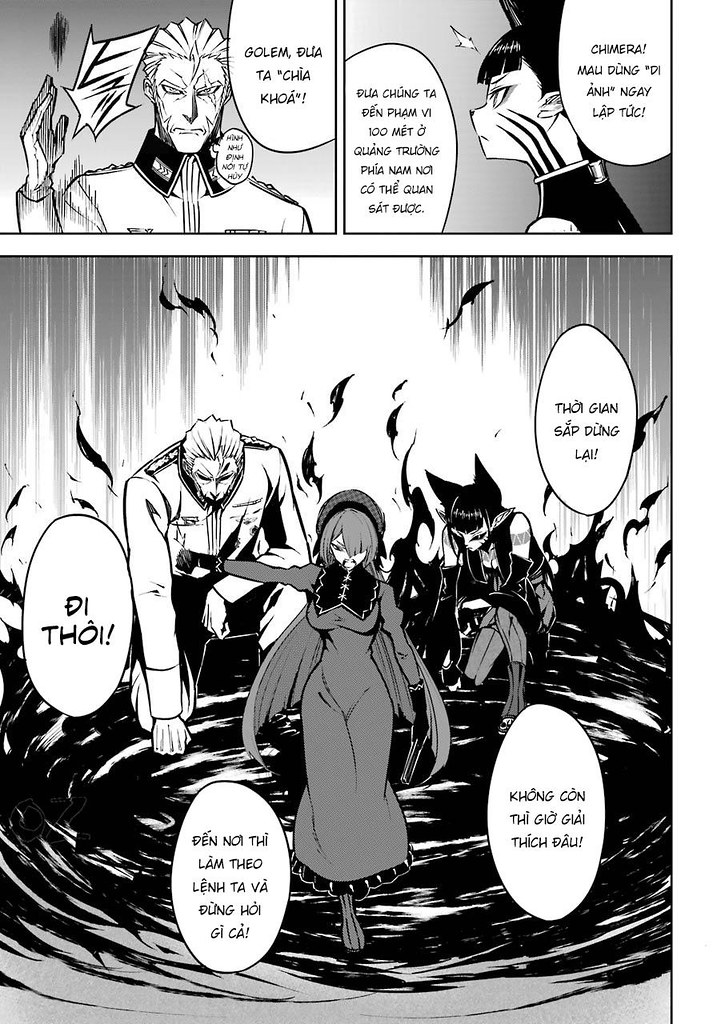The black-and-white cartoon is a detailed comic book page divided into three main panels. The top section consists of two landscape-oriented rectangles. In the top left panel, a man is shown from the chest up, wearing a military-style uniform. He appears to be tossing a piece of paper into the air, with two conversation balloons beside him filled with text in what appears to be Vietnamese, suggested by the numerous accents and diacritical marks typical of the language. The top right panel features a female figure with cat-like characteristics, including whiskers and black hair with bangs. She is shown in profile, facing left, with conversation balloons on either side in the same foreign language.

The bottom half of the page is a larger, portrait-oriented scene. At the center stands a woman dressed in a long gray gown with a black collar, long hair, and a headband. She has one arm outstretched dramatically. Behind her, the man from the top left panel and the cat-like female from the top right panel are kneeling, bowed down as if in submission or supplication, amid swirling black flames. The composition features four more conversation balloons in Vietnamese, two on each side of the panel. The entire illustration is rendered in a black-and-white line art style, with a photographic representationalism approach, giving it a very detailed and expressive look.